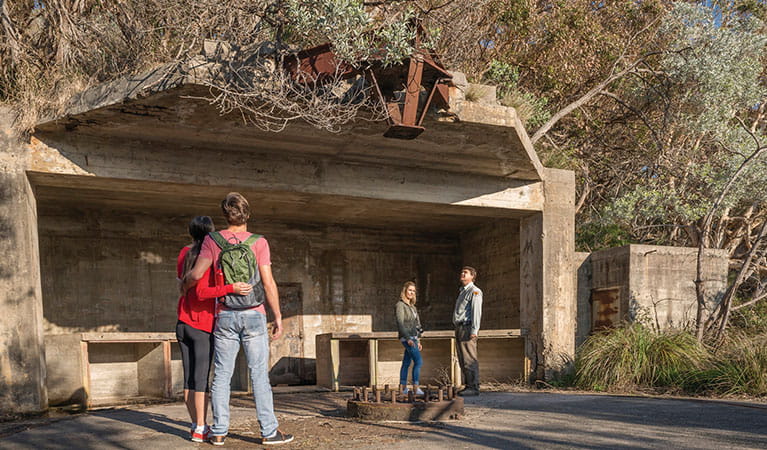In this color daytime photo, we see four people standing in front of an abandoned structure, possibly a modern-day doomsday bunker or a damaged heritage site. The background is filled with a mix of green and dead trees under a clear blue sky, highlighting the sunny ambiance. The structure itself, carved out from the side of a mountain or hidden beneath trees, is primarily made of two-foot thick concrete walls and ceiling, with additional stone elements hinting at its robustness. However, the bunker is now exposed to the elements, its front wall collapsed and various parts overgrown with plants and bushes.

The partially intact roof features a metal contraption protruding from its center, and inside, remnants of counters and stone inscriptions are visible against the back and side walls. There is even a glimpse of some designs and patterns on the walls. Standing around this structure are four individuals: two couples. One couple, standing to the left with their backs to us, consists of a man in jeans and a pink t-shirt with a green backpack, and a woman in a red jacket, black quarter pants, and red shoes. He has his arm around her, and she reciprocates with her hand behind his back. The other couple, at the center of the image, faces the camera. The woman here is also wearing a red jacket and blue jeans, with blonde hair. The man beside her is in a blue shirt and gray pants, looking upwards intriguingly. Amidst the ruins, the grown vegetation, and the human presence, this image captures a scene that blends nature, decay, and human curiosity.